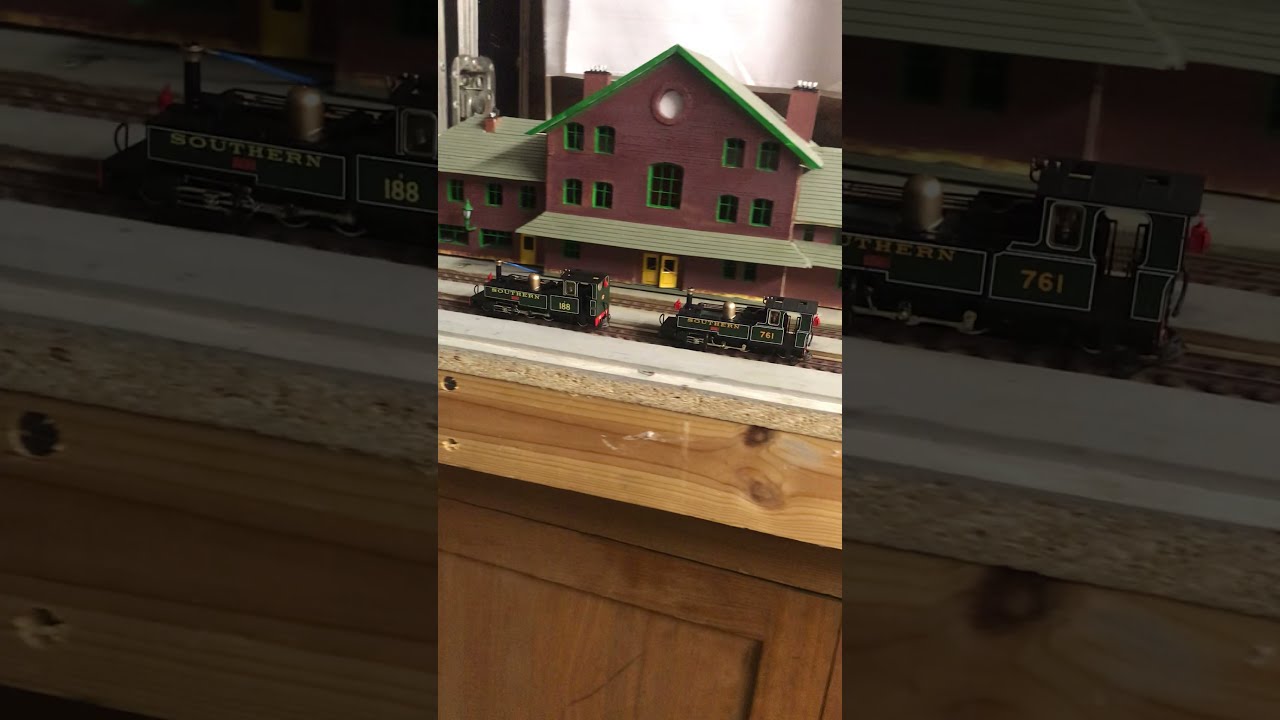The image showcases an intricate model train set placed on a brown surface, possibly a cabinet or table. Central to the scene are two vintage-looking train engines labeled Southern 188 and Southern 761, both in motion on parallel tracks. These trains are navigating a circular loop, but only a segment of their journey is visible. In the background stands a red brick building with yellow doors at the base, a green roof, and green-framed windows, resembling an old-fashioned train station. The collage of images includes a main wide shot and additional close-up views of the trains on the track, highlighting the detailed craftsmanship of the model set.